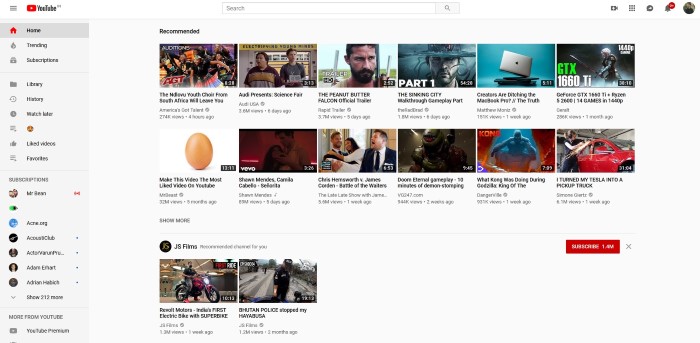A detailed screen capture of a desktop computer displaying a YouTube web page. In the upper left corner, the YouTube logo is prominently featured, consisting of a red rectangle with a white play arrow. Centrally positioned at the top of the screen, there is a search text box. On the left side of the page, a vertical sidebar presents various YouTube menu options. Among them, the "Home" option, depicted with a red house icon, stands out, highlighted in a gray bar, indicating it is the selected menu. The page itself has a clean, white background, showcasing an array of recommended videos. There are three distinct rows of video thumbnails: the top and middle rows each display six videos, while the bottom row features only two.